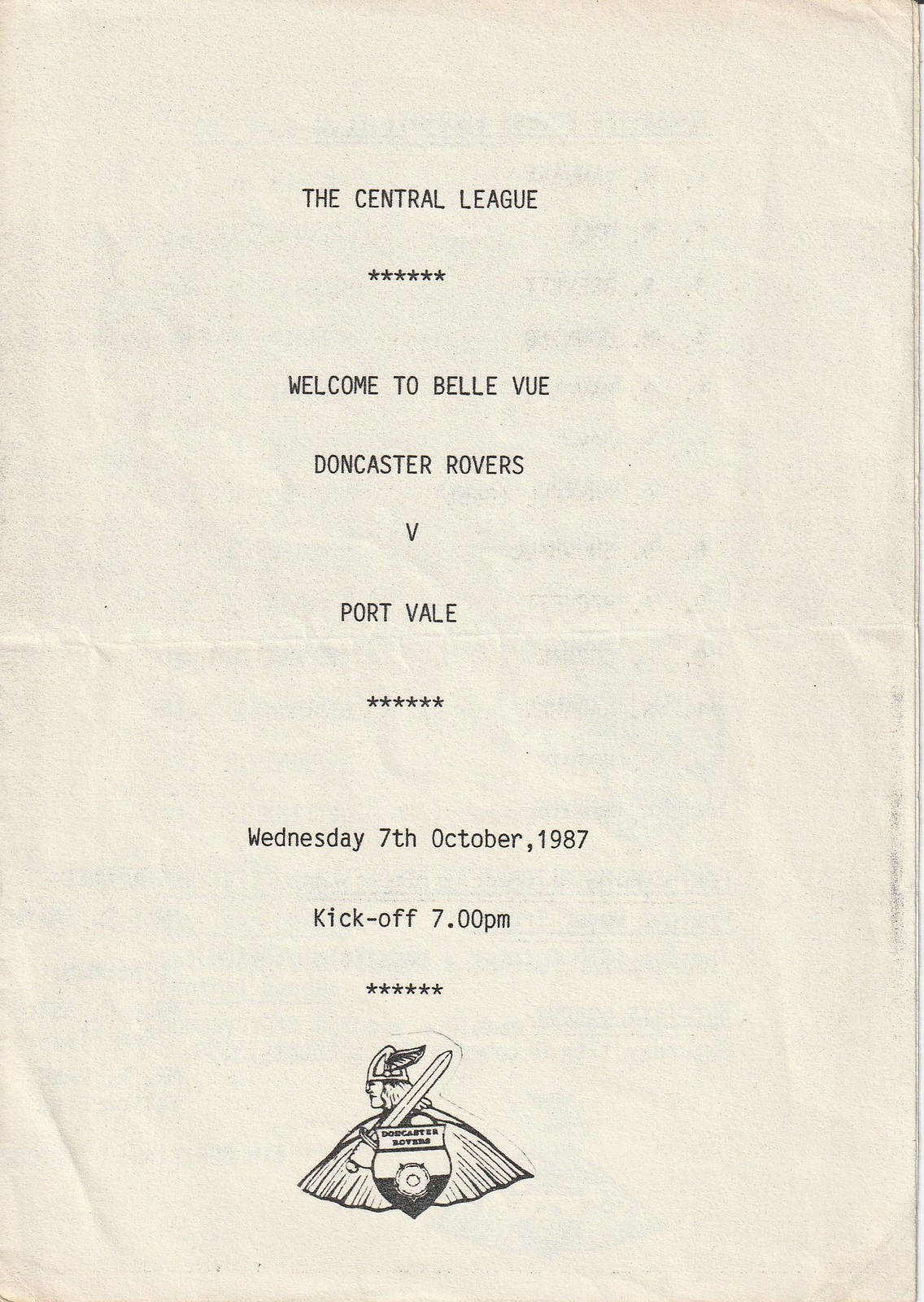This image showcases a vintage, yellowed program page from a soccer match within the Central League featuring Doncaster Rovers versus Port Vale. The text is typewritten in bold, black letters, predominantly in all caps. It reads "THE CENTRAL LEAGUE" at the top, followed by a row of asterisks. Below that, it welcomes spectators to Bellevue and mentions the match between Doncaster Rovers and Port Vale. Another row of asterisks separates this from the match details, which state: "Wednesday, 7th October 1987, Kickoff 7 PM," followed by yet another row of asterisks. The page is visibly wrinkled, indicative of its age. At the bottom of the page, there is a detailed graphic of a Viking holding a sword, adorned in a robe and helmet with wings, alongside a shield inscribed with "Doncaster Rovers," representing the club's logo. Faint text is discernible through the paper, suggesting additional information, likely team rosters, on the reverse side.